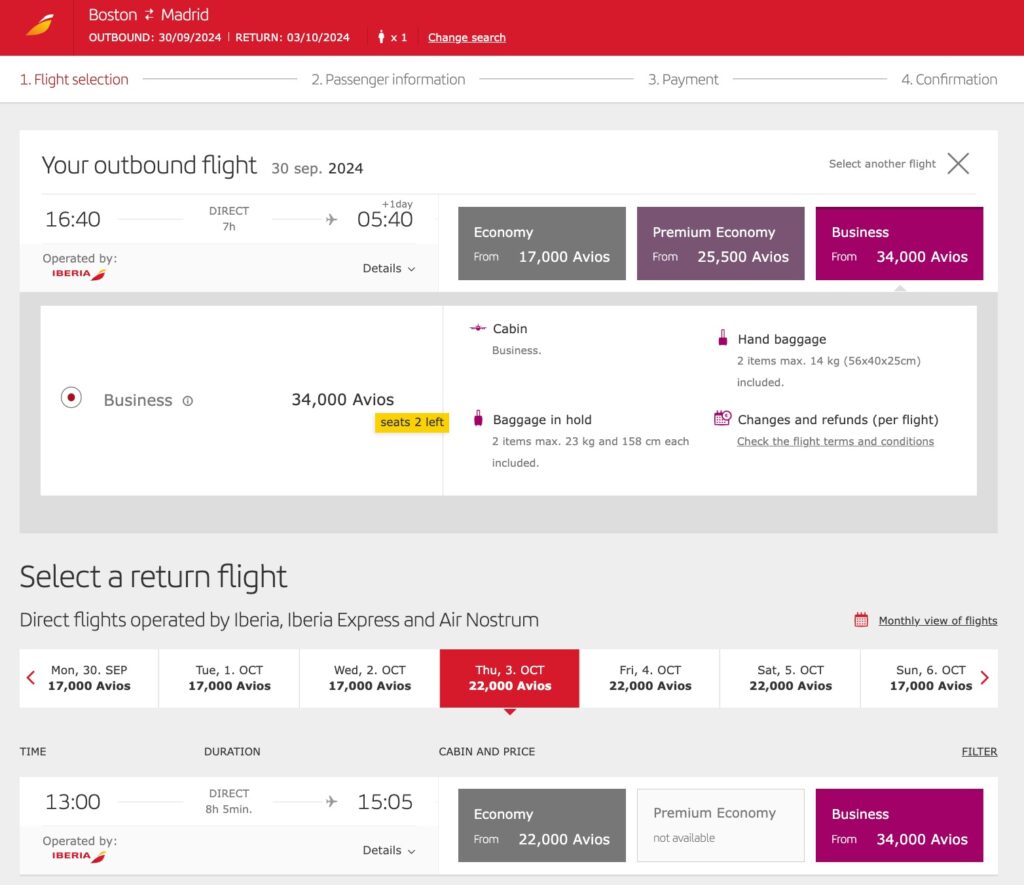The image depicts a flight booking interface for a trip from Boston to Madrid. In the top left corner, there's a header displaying "Boston to Madrid" alongside a wing-shaped logo. Directly below, the words "Outbound" are stated, followed by the date "30/09/2024." Adjacent to this is the "Return" date, noted as "03/10/2024." An icon representing a single traveler is also visible, denoted by "x1" beside a person symbol.

Below this section, a progress bar illustrates the booking process through numbered steps: "1. Flight Selection," "2. Passenger Information," "3. Payment," and "4. Confirmation," with a line connecting each stage.

In the middle left of the interface, a boxed section provides details about the outbound flight on "30 September 2024," which departs at "16:40" for a direct journey lasting "7 hours and 05 minutes," arriving the next day at "05:41." To the right of this information, three options for seat classes are displayed, each with their respective Avios points: "Economy" for 17,000 Avios, "Premium Economy" for 25,500 Avios, and "Business" for 34,000 Avios.